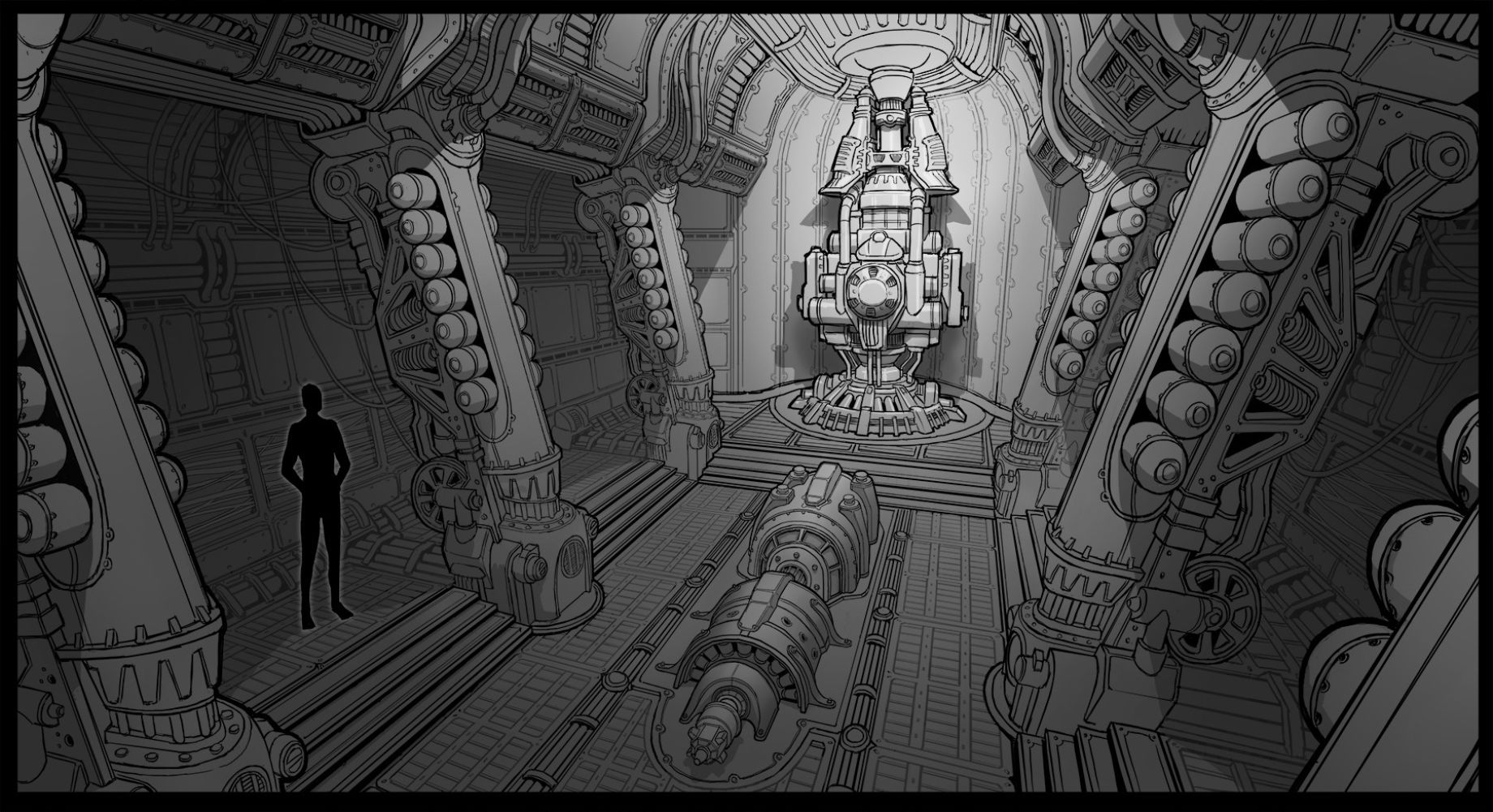The black and white image appears to be a detailed, cartoon-esque drawing of a futuristic and mechanical interior, possibly the inside of a sophisticated machine or ship. The scene features clean lines and varying shades of gray, aside from a stark black shadowed figure on the left or right, adding a mysterious presence to the room. The figure stands amidst a complex environment, surrounded by six slanted pillars, each adorned with intricate mechanical components.

Dominating the central portion of the image—set further back—is a prominent circular device, likely the core or control center of the machine. This device is interconnected with a web of wires, pipes, and cables, suggesting it could be the main power source or the brains of the apparatus. Surrounding this focal point, the room contains various wheels, tanks, and cylinders, all contributing to the intricate, almost industrial aesthetic. This visually rich scene, illuminated by a bright spotlight on the central device, evokes the feeling of being inside a highly advanced and enigmatic piece of technology.